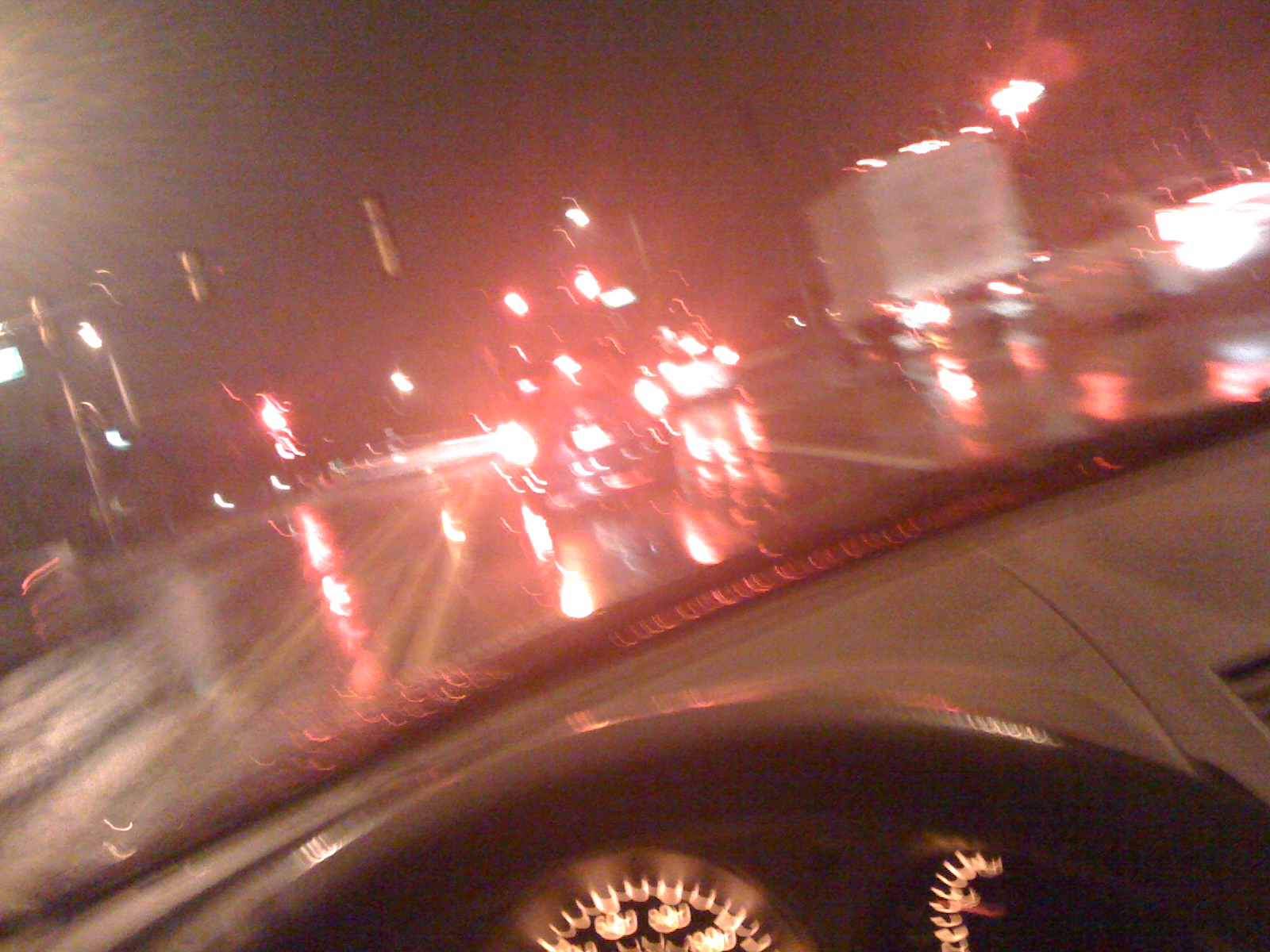The image is a blurry, out-of-focus photograph taken from the inside of a car, peering over a dark gray steering wheel and a lighter gray dashboard. The photo, tilted slightly to the right, reveals illuminated driver instruments, including part of the speedometer and fuel gauge, in the bottom center of the frame. Through the rain-slicked windshield, a rainy city night is observed, with numerous bright red brake lights and stoplights glowing in the scene. In front, a small car has its brake lights on, likely stopped at a traffic light, while on the right, a larger box truck is seen without active brake lights. To the left, there are street poles holding traffic signals for the opposite lane, which appears empty. The night sky is pitch black without any visible stars, contributing to the overall glistening and shiny appearance of the wet road and lights.